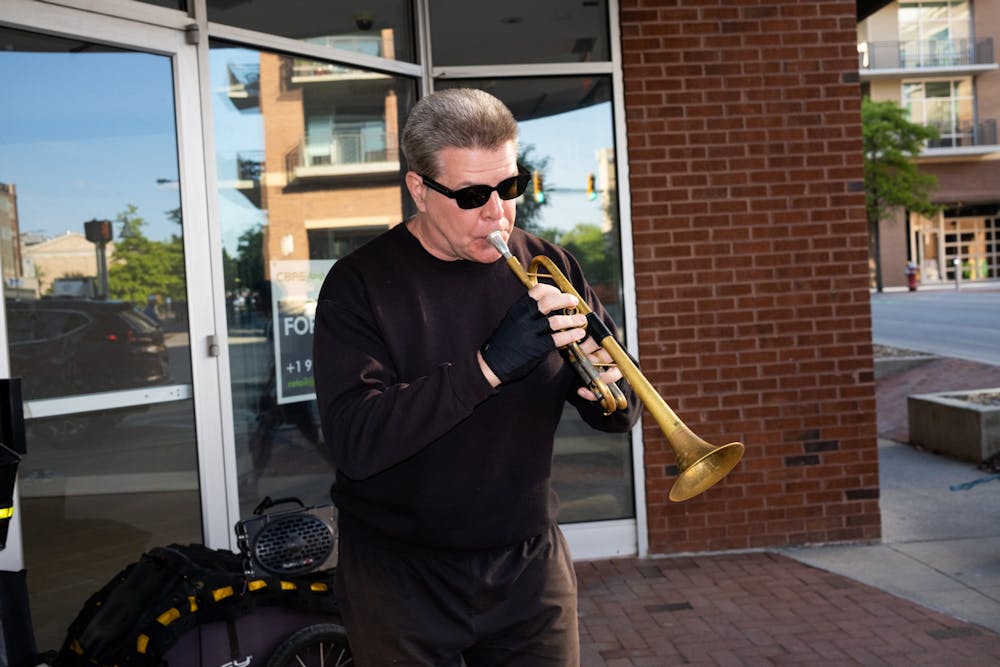A man, dressed entirely in black with a black sweatshirt, black joggers, black fingerless gloves, and black sunglasses, is playing a gold trumpet in front of a building entrance. The building features a mix of glass doors and brick walls, with the entrance partially framed by brickwork in shades of red and black. Behind him, positioned to his left, is a small amplifier, while to his right and farther back is a glass storefront and a sidewalk area. The glass panes reflect nearby buildings, cars, and trees. The major colors in the photo include black, gold, white, green, and various shades of brown and gray. The scene captures a mix of urban elements including brickwork, glass, and hints of greenery in the distant reflections.